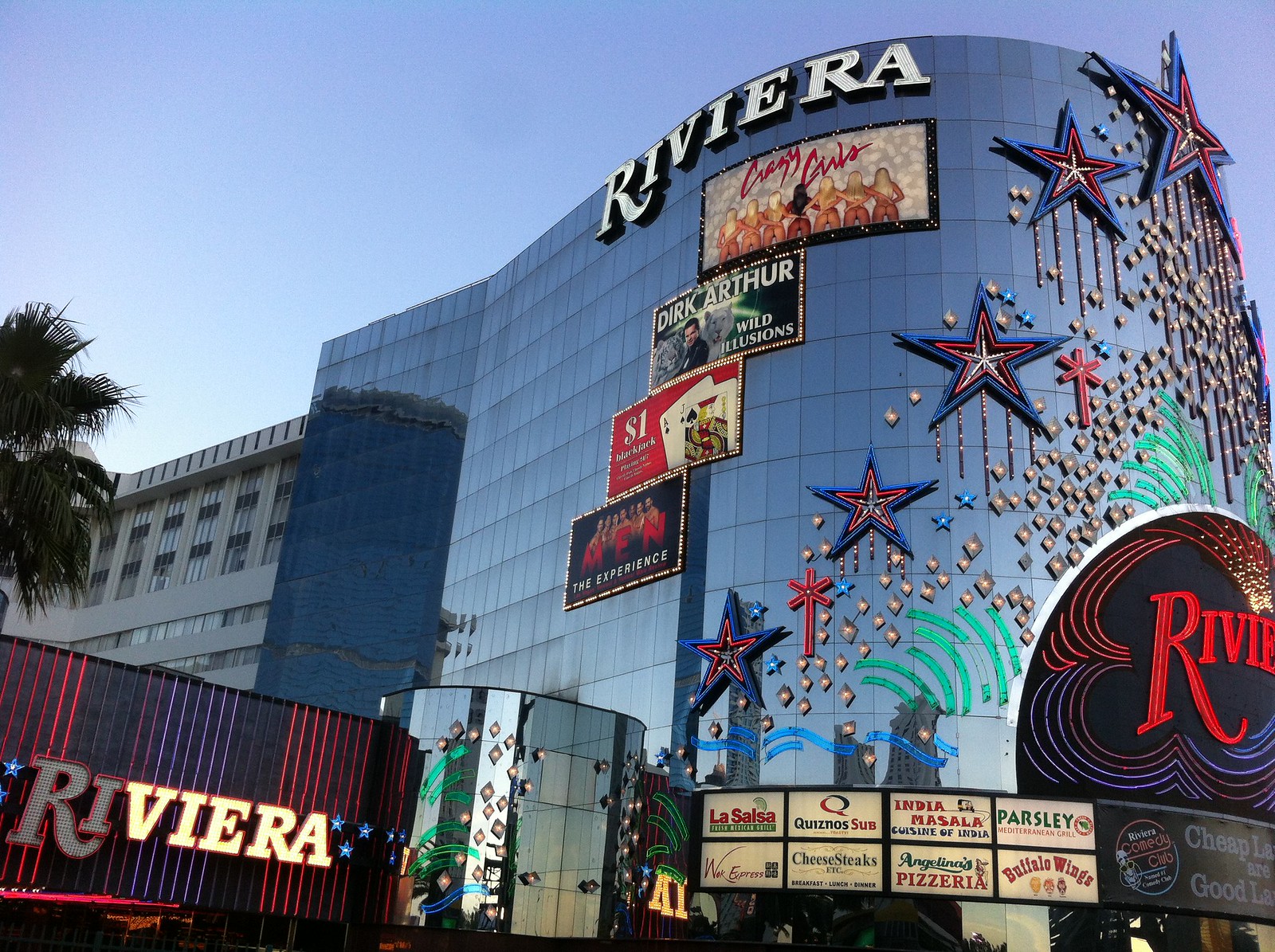This photograph captures a tall, glass-walled building along the Las Vegas Strip, prominently displaying the name "Riviera" in bright red letters. The façade of the building is adorned with giant, illuminated stars in red, white, and blue, which contribute to its vibrant nighttime appearance. The sky above is a clear, pure blue with not a cloud in sight, enhancing the daylight setting of the image. 

On the building, numerous large signs advertise a variety of attractions and businesses. Prominent posters include headliners like "Crazy Girls," a male revue, "Dirk Arthur Wild Illusions," and mentions of comedy and magic shows. Additional billboards at the bottom highlight an array of dining options including Quizno Subs, Buffalo Wings, Cheese Steaks, La Salsa Fresh Mexican Grill, India Masala Cuisine of India, Parsley Mediterranean Grill, Wok Express, and Angelina's Pizzeria, catering to breakfast, lunch, and dinner needs.

A palm tree is positioned toward the left-center of the image, which frames the Riviera building alongside adjacent hotels. The building surfaces glisten in shades of light blue, silver, grayish-blue, and tan, enhanced by a multitude of sparkles and colorful lights spread across the structure. The setting encapsulates the bustling and eclectic essence of Las Vegas, making for a visually arresting scene.